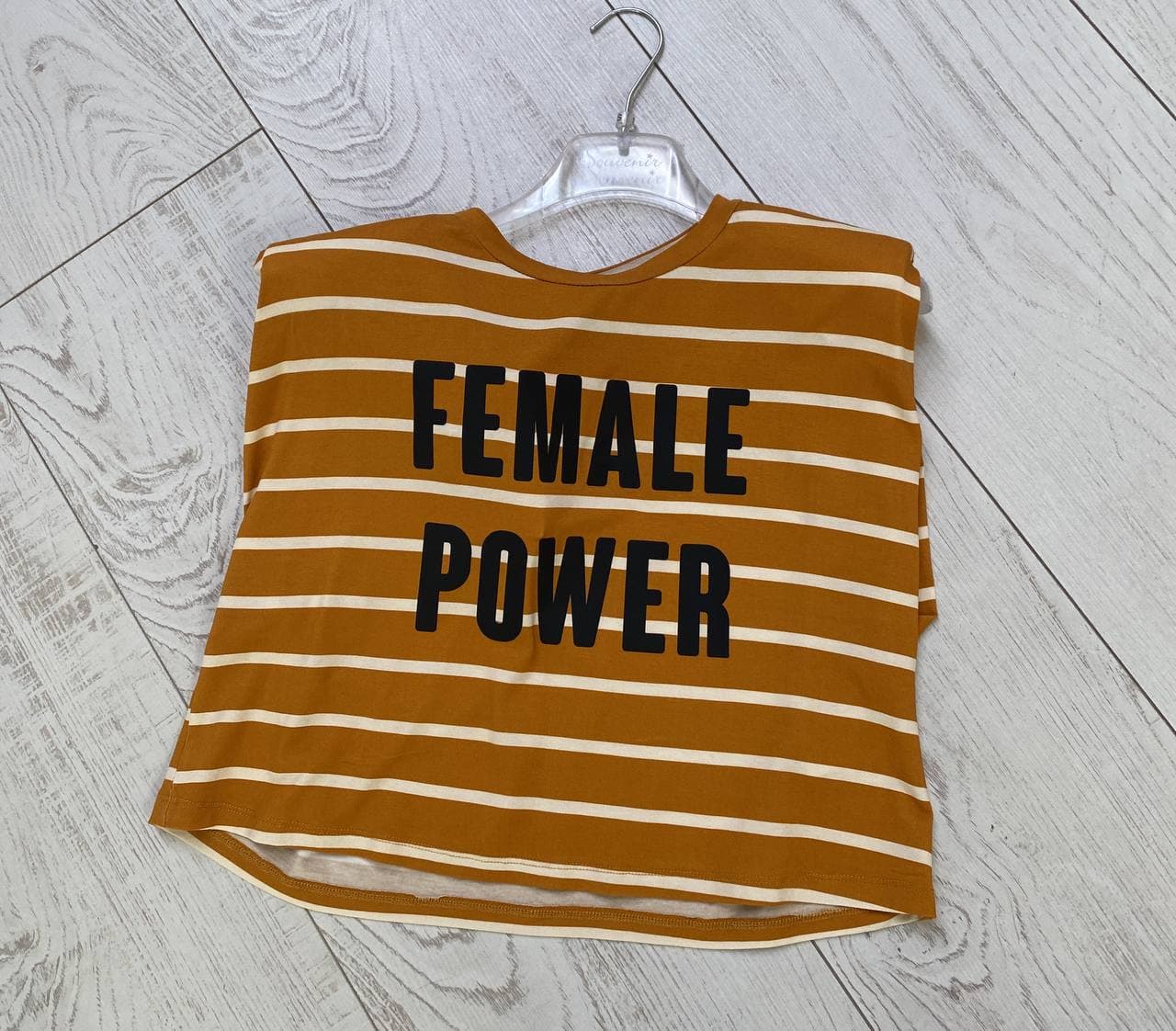The image features a t-shirt on a plastic hanger with a metal hook, positioned on a gray kitchen table. The shirt prominently displays the phrase "Female Power" in bold black letters. It has a design of horizontal yellow and white stripes and resembles a crop top, complete with sleeveless arms. The table's surface consists of light gray wood planks arranged diagonally, with darker gray lines highlighting the gaps and grain patterns in the wood.